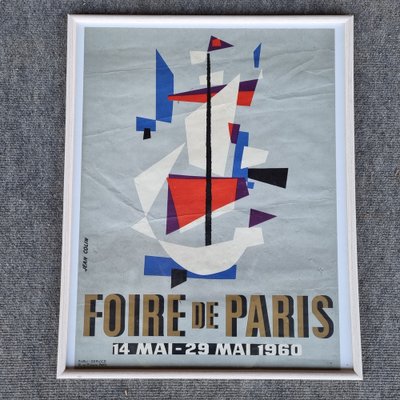The poster has a light gray, slightly crinkled background and is bordered by a white picture frame. At the center are various abstract shapes in blue, red, purple, and white, including triangles, trapezoids, half-circles, and an obscure U-shaped form that resembles an abstract boat. Running vertically through the middle of the composition is a black line, topped with a small purple flag. Below the central image, in elegant goldish-brown letters with a black shadow, the text reads “FOIRE DE PARIS.” A black banner at the bottom features the dates “14 MAI - 29 MAI 1960” in white lettering. The entire artwork is set against a fabric-like gray background with some white detailing and definitive lines running across it.